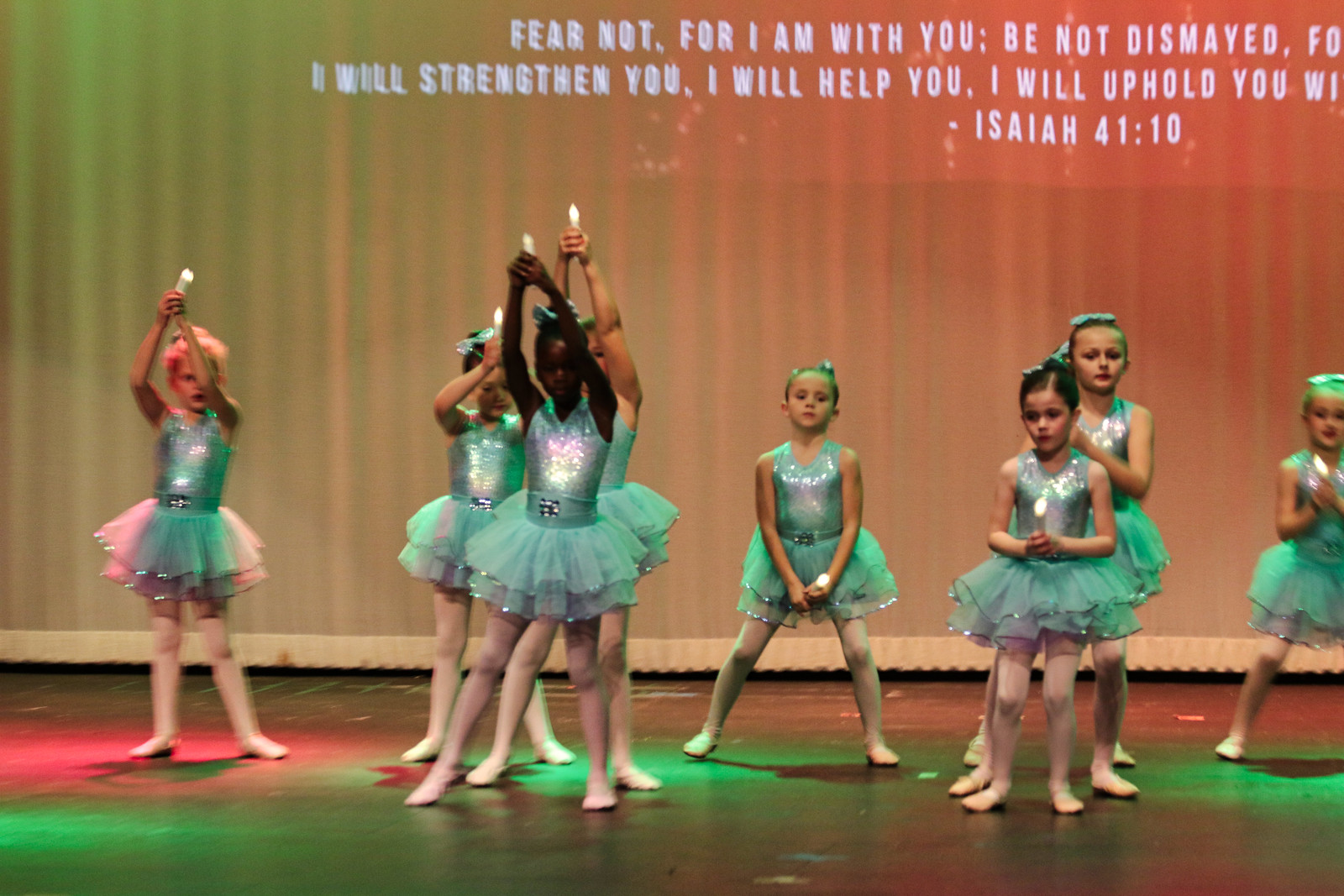The image depicts a stage adorned with green and red lighting, featuring a group of nine young ballerinas, around six years old, dressed in green tutus, white stockings, and ballet slippers. They are holding lit candles and arranged in a line, performing various dance moves. The backdrop consists of a white curtain illuminated by a pinkish hue, with a projected religious text that reads, "Fear not, for I am with you. Be not dismayed, for I will strengthen you. I will help you. I will uphold you…" The quote is partially cut off, and it is sourced from Isaiah 41:10. Among the girls, there is a notable diversity, including one black girl, highlighting the inclusive nature of the performance. The scene captures a religious-themed ballet recital, emphasizing unity and faith.